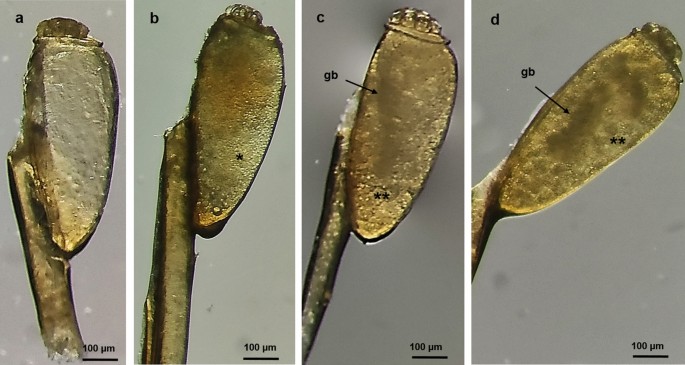This professional, full-color horizontal image is divided into four individual microscopic images, each measuring 100 micrometers, which is beyond the resolution of the human eye. These images are arranged with a white border separating them, set against a gray background. Each image is labeled in the upper left corner as A, B, C, or D. The main subject in all four images is a brown, irregularly shaped object resembling either a cell or a flat, vegetative structure attached to a stalk. Each image is detailed with labeling in the bottom right corner indicating the 100 micrometers scale. In images C and D, an arrow marked "GB" points to specific parts of the object, enhanced by two digitally added black stars for emphasis. The object’s appearance is somewhat translucent with possible crystalline formations along the stalk, contributing to its shiny and clear look.